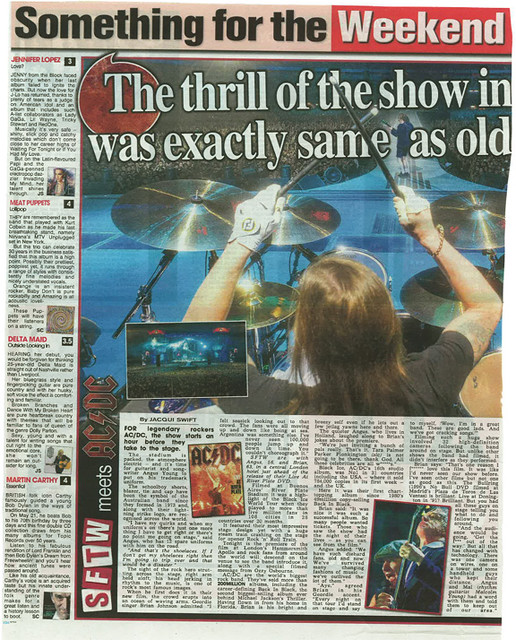The image is a newspaper page with the top heading reading "Something for the Weekend" where "Weekend" is highlighted in white text within a red box. The main headline beneath the heading is partially cut off but reads "The thrill of the show in... was exactly the same as old..." The page features a large central photo showing a drummer viewed from behind, playing on a stage with a lead guitarist towards the front, right near a ramp leading into what appears to be a large audience. The photo captures a concert setting with visible, though indistinct, spectators. The left column of the newspaper lists various small stories about different artists such as Jennifer Lopez, Meat Puppets, Delta Maid, and Martin Carthy. The main article spans four columns of text, though the font is too small to read. Within these columns, there are additional smaller photos, including one labeled "ACDC" featuring people, and another showing a person singing into a microphone with a guitarist in the foreground. A tiny panoramic photo of the stage is also overlaid in the lower left-hand corner of the main concert photo.